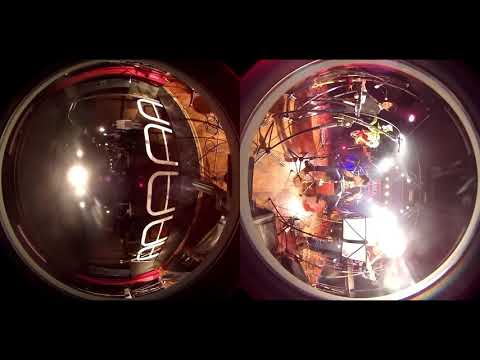The image comprises two circular and slightly tilted sections, each providing a distinct yet connected view of a dimly lit stage setup. The left image, skewed 90 degrees to the left, primarily displays a dark area with a potential curtain backdrop. A white guardrail is visible in the front, suggesting a stage setting. The lower portion, around 20%, reveals a wooden floor, and faint outlines of stage equipment hint at a setup in progress. The right image, tilted 90 degrees to the right, shows a more complete stage scene with a wooden floor and a man centered, playing the drums. To his left, another performer stands on a raised platform with a microphone, presumably playing a keyboard. Bright lens flares obscure parts of the background, creating a luminous, hazy effect, and additional equipment like music stands can be faintly seen. Overall, both circular images exhibit a concert-like atmosphere with a strong emphasis on stage lighting and musical performance.